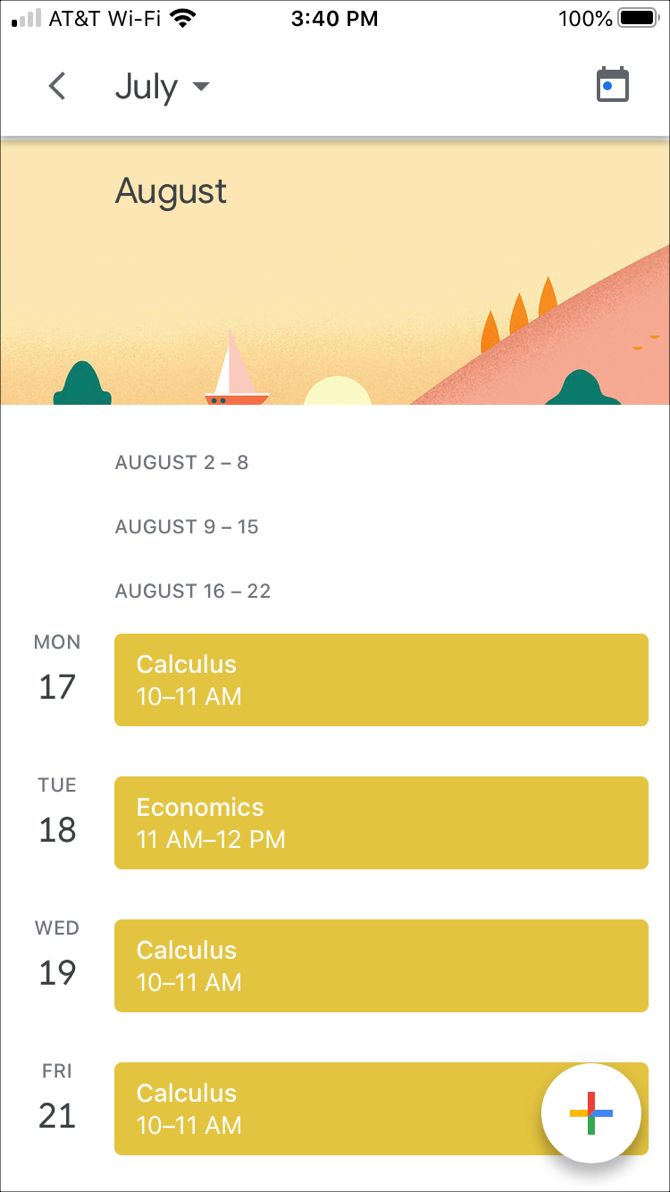This screenshot captures a smartphone display detailing a weekly calendar schedule. At the top, various status indicators are visible: a strength bar with one black and three gray lines, an AT&T carrier label, a Wi-Fi symbol, a network fan icon in black, the time marked as 3:40 p.m. in black font, and a battery indicator showing 100%.

Directly beneath this is a navigation line featuring a back arrow, the month "July" accompanied by a downward-facing triangle, and on the far right, a calendar icon marked with a blue dot.

Below this is a header titled "August" set against a vibrant background depicting peach-colored mountains, orange-hued trees, and two additional bushes. This section transitions into the detailed calendar dates, listed as:
- August 2nd to 8th
- August 9th to 15th
- August 16th to 22nd (this particular range is in gray, likely indicating the current week or a specific emphasis)

The detailed schedule includes the following entries, each highlighted with a gold bar:
- Monday, August 17th: "Calculus" from 10 to 11 a.m.
- Tuesday, August 18th: "Economics" from 11 a.m. to 12 p.m.
- Wednesday, August 19th: "Calculus" from 10 to 11 a.m.
- Friday, August 21st: "Calculus" from 10 to 11 a.m.

In the lower right-hand corner of the screen, there is a multicolored round icon divided into four sections with the colors yellow (left), blue (right), green (bottom), and red (top).